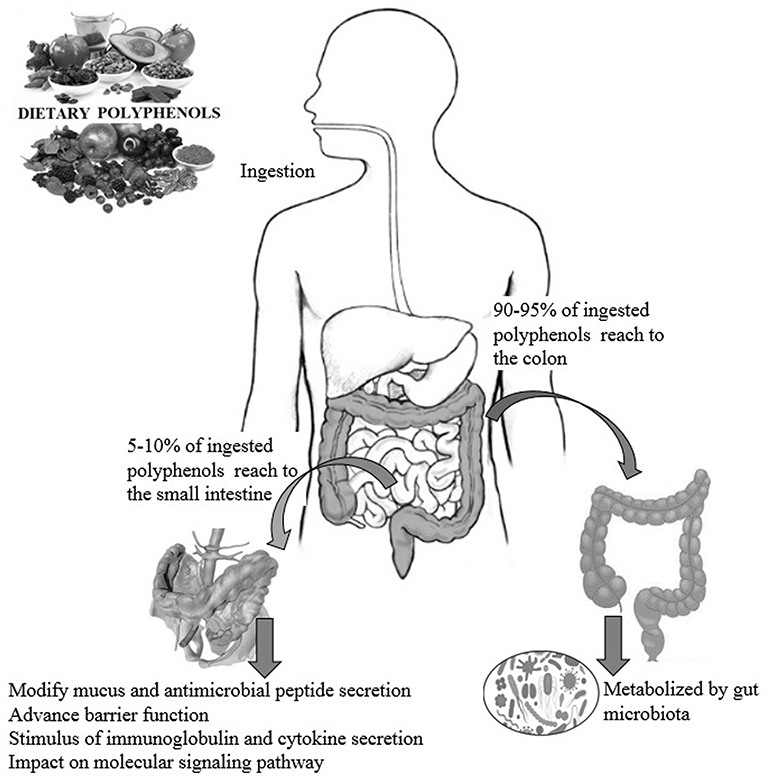The image is a detailed scientific diagram focused on the digestion of dietary polyphenols and its impact on gut health. In the upper left corner, there's a graphic featuring various foods with the label "dietary polyphenols." To the right, an outline of a human figure is depicted, facing left, illustrating the digestive system, from the mouth through the esophagus down to the stomach and intestines. The process starts with the label "ingestion" by the mouth. Text on the right states that 90-95% of ingested polyphenols reach the colon, accompanied by an arrow pointing to the colon area, noting that these polyphenols are "metabolized by gut microbiota."

On the left side, it's noted that 5-10% of ingested polyphenols reach the small intestine, with an accompanying arrow pointing from the small intestine to descriptive text below. This text outlines the subsequent effects: modification of mucus and antimicrobial peptide secretion, enhancement of barrier function, stimulation of immunoglobulin and cytokine secretion, and impact on molecular signaling pathways. The entire illustration is rendered in black, white, and shades of gray, emphasizing the anatomical details and the flow of polyphenols through the digestive system.